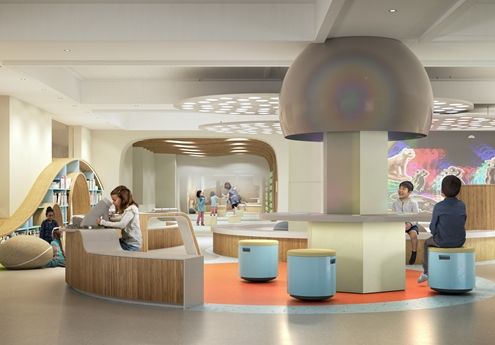The image depicts a spacious, well-lit room characterized by a white ceiling and walls. At the right side, a column with a domed top supports the ceiling. Surrounding the column is a small table with round blue stools. Several children are present: one child sits on a blue stool on the far right, and another child is seen in the background. In the foreground, a woman is seated at a desk, seemingly assisting children. One child nearby appears to be looking through something. Additionally, the room features blue seats and a floor with a prominent orange circle integrated with some tan areas. Some tables have wooden fronts, contributing to the room's warm and functional ambiance. On the left side, there's a low counter where a girl sits, facing left. In the background, another room with more people can be observed. The overall atmosphere is bright and inviting, suitable for a variety of activities.